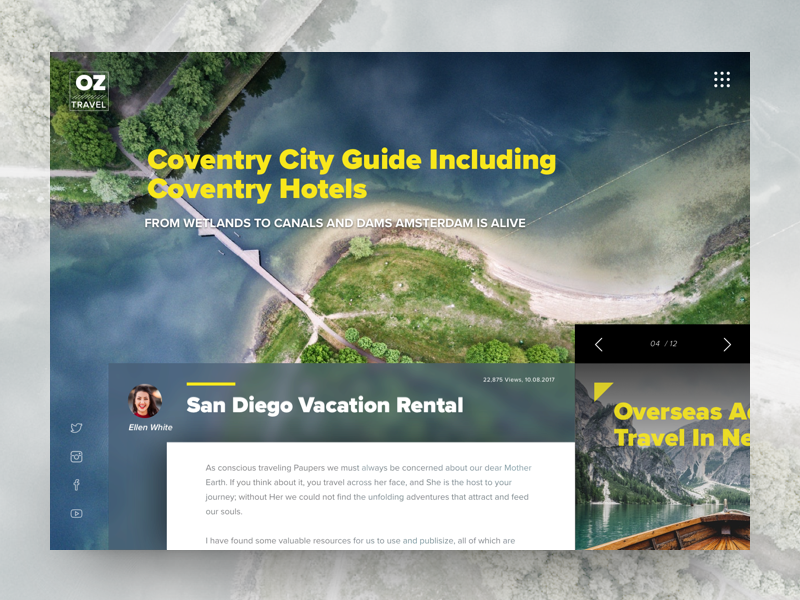A drone or airplane has captured a stunning aerial view, presenting an expansive and detailed scene. The primary landscape showcases a pristine, white sandy beach juxtaposed against the deep blue hues of the sea. The vibrant greenery contrasts vividly with the stark, uninhabited appearance of the land. A lonely bridge connects two islands, devoid of any cars or people.

Interestingly, superimposed upon this image is a series of digital overlays. A prominent one reads "Coventry City Guide," promising insights into Coventry hotels, alongside other features. Despite this, the actual visuals seem far removed from urban life, emphasizing nature's untouched beauty instead.

Amidst these overlays, a pop-up box advertises a "San Diego Vacation Rental," complete with a profile picture of a person named Ellen White and a brief write-up in a separate white box. To the side, another cut-off box mentions "overseas... travel in NE," illustrated with an image of a wooden boat gliding through the sea.

Towards the top left corner, the text "Oz Travel" appears, while on the right, a cluster of small dots can be seen. This collage of colorful overlays stands out distinctly against a neutral gray backdrop, adding layers of intrigue to the already captivating aerial photograph. In the distance, high mountains with snowy peaks loom, further enriching the scenic panorama.